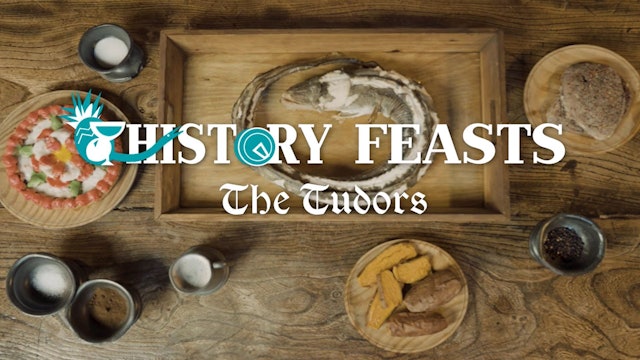The image is an overhead view of a rustic wooden table set for an event titled "History Feasts: The Tudors," showcased in bold white text with a subtle teal-accented logo featuring a pineapple and martini glass. Central to the image is a wooden serving board displaying a long, slimy fish, possibly an eel, steamed or poached. Surrounding the main dish, various wooden plates hold an assortment of food: sliced sweet potatoes, a meat patty, and an indiscernible red dish. Scattered across the table, hand-thrown pottery dishes contain herbs, peppercorns, and other seasonings, enhancing the medieval feast ambiance. There are also cups filled with a white beverage and a decorative floral pastry or salad, contributing both to the historical theme and the artistic presentation.